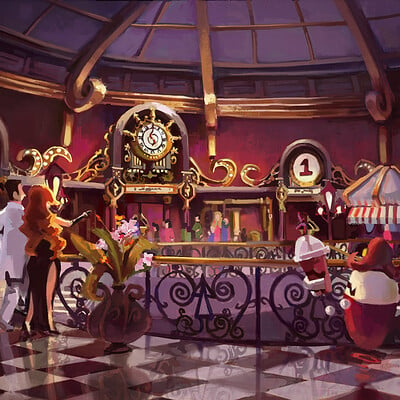In this animated Disney movie scene, the setting is an elegant, domed indoor hall illuminated by a night sky barely visible through the tall, glass ceiling. The floor is distinctively patterned with red and white checkers. Dominating the scene is a finely wrought, black iron railing hinting at a balcony overlook. To one side, a large potted plant with a face on its pot and fern-like leaves stands prominently, adding a quirky touch.

Center stage, a striking woman with long, flowing red hair, dressed in a sleek black gown featuring slits up the side, is captured pointing towards something off-screen. She wears high heels and is accompanied by a man in a crisp white tuxedo with dark brown hair. Their expressions are filled with curiosity and intrigue as they walk deeper into the hall.

To the right of the couple, an obese girl, almost cartoonish in appearance, holds a red drink cup with a white lid and straw, resembling a slurpee. Above them stands a grand clock, intricately designed with a white and beige face, black Roman numerals, and a golden sun-like border.

In the background, you can see another group of people approaching, possibly ascending from elevators, adding to the sense of movement and depth in this richly detailed, animated scene.